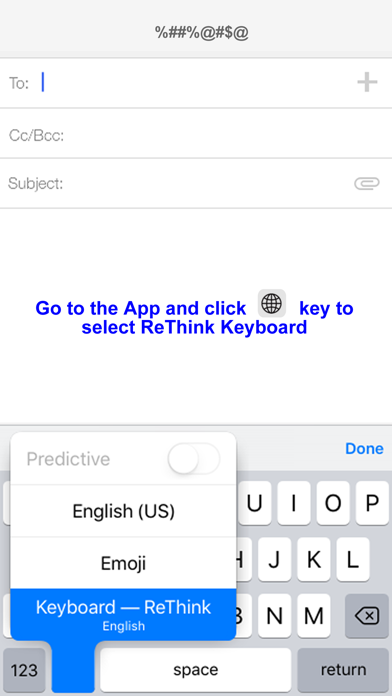The image depicts a screenshot taken from a cell phone displaying an email composition screen. At the top of the image, a gray rectangle contains a string of characters: "%##%@#@$@" which may be a placeholder or code. Below this, the screen shows the "To:" field followed by a blinking blue cursor, indicating where the user can enter the recipient's email address. Adjacent to this is a plus sign, likely for adding additional recipients. 

A faint gray line separates the "To:" field from the next section, which shows "CC/BCC:" also followed by a colon and a blank field for additional email addresses. Continuing downward, the "Subject:" field appears, also empty, with a paperclip icon on the right side symbolizing an attachment option. 

In the body of the email, instructions are displayed: "Go to the app and click the world icon to select the Rethink Keyboard." Further down the screen, the existing text reads "Keyboard Rethink," indicating the selected keyboard type. The entire screen is segmented by faint gray lines, guiding the user's eyes through the structured layout of the email composition interface.